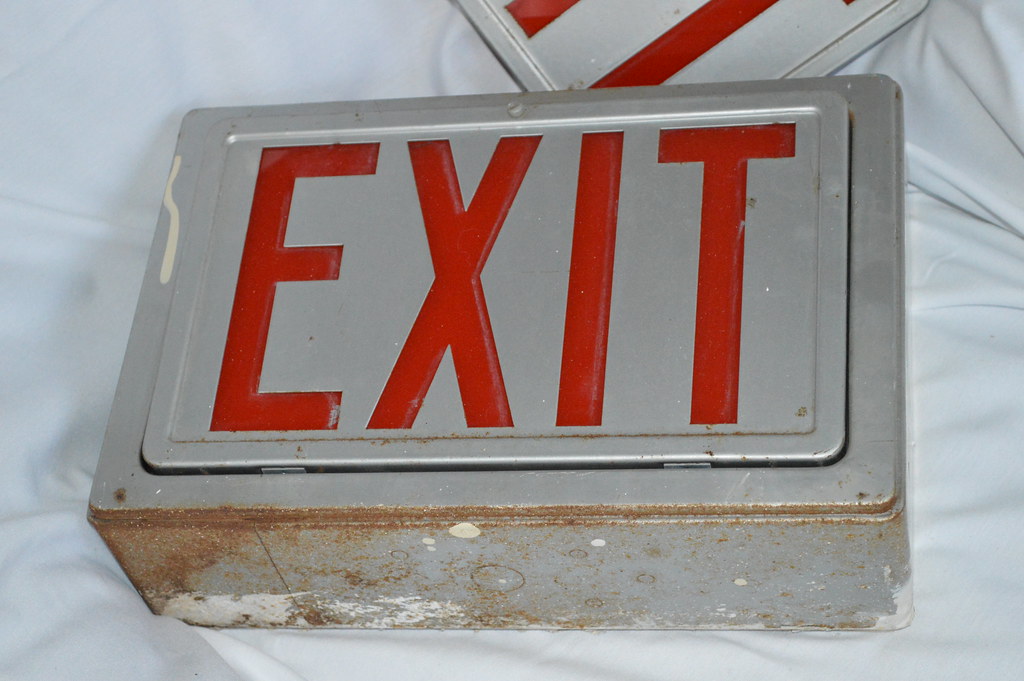This close-up photograph captures an old, slightly rusted exit sign lying flat on a somewhat crumpled white sheet that takes up the entire background. The exit sign, made of gray metal, prominently displays bright red, block capital letters spelling "EXIT" on its faceplate. This main subject, detailed with minor rust at the bottom and white paint splatters dripping down the left side, hints at its age and previous use. Directly behind the exit sign in the upper part of the image, there's a portion of another sign with indistinct red stripes, likely letters, yet too obscured to identify fully. The white sheet beneath, dotted with minor folds and creases, enhances the textural contrast in the image.